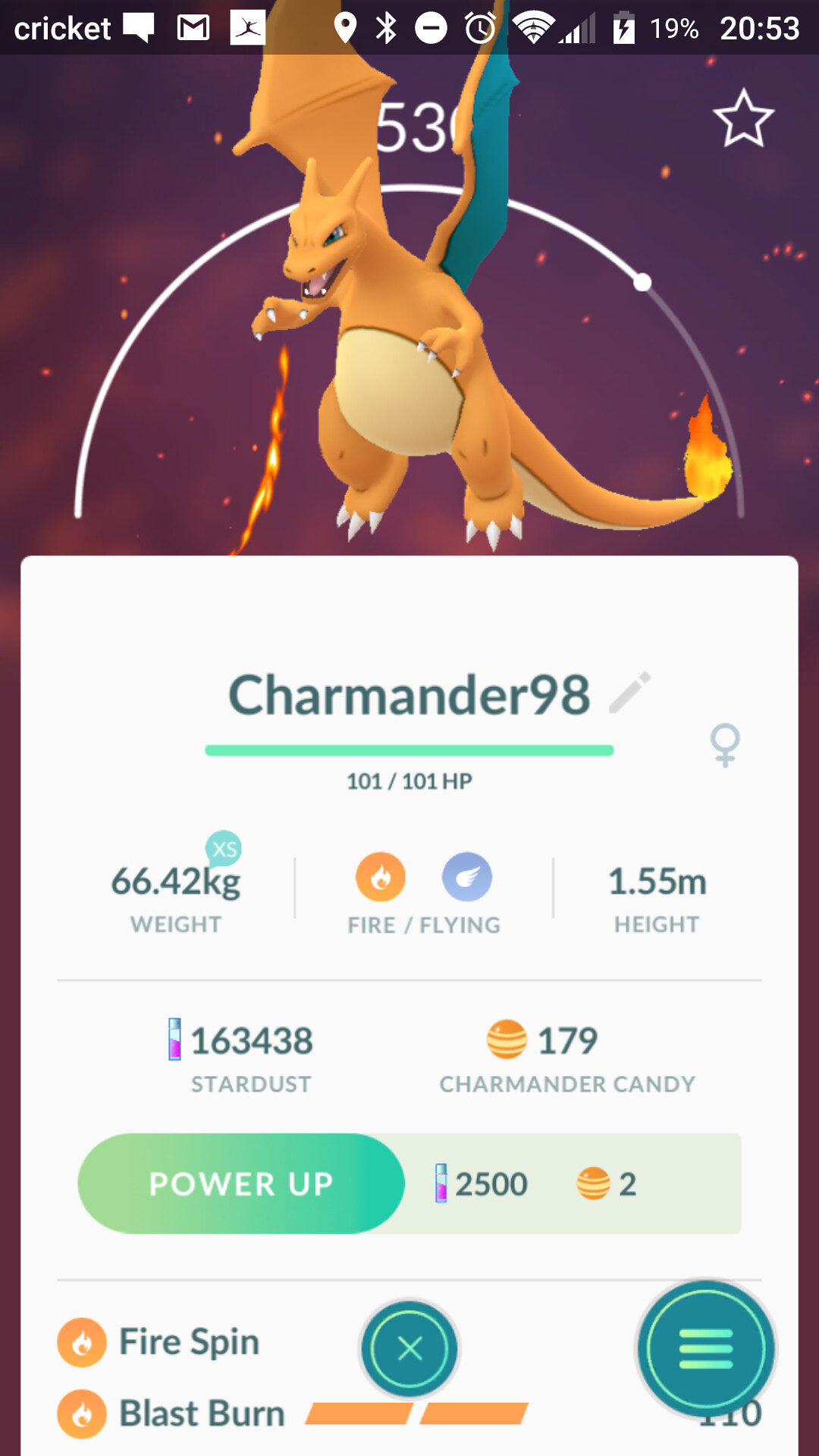This image is a detailed color photograph capture of a cell phone screenshot, depicting an app game focused on the Pokémon character, Charmander, notably labeled as Charmander98. Displaying cell service at the top left with the word “cricket,” it indicates a battery life of 19% and the time as 20:53. The central figure, Charmander, is a dragon-like creature with light orange-brown skin, sharp teeth, big claws, and striking blue eyes. Notably, the dragon has blue-tinted undersides to its wings and a flame at the end of its tail, along with another flame being thrown from one paw. Charmander is set against a striking dark purple background, accentuated by a white ellipse and a star in the top right. Technical details below the character reveal measurements of 66.42kg in weight and 1.55m in height along with 163438 Stardust. The interface displays a conspicuous green “Power Up” button on the left and continues with further game-related statistics and navigation aids like an orange bar graph labeled “fire spin” and “blast burn.”